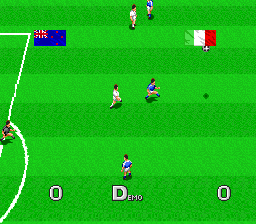This image is a square screenshot capturing the nostalgic essence of an old-school, pixelated video game focused on soccer. The graphic style is distinctly vintage, characterized by its simplistic, 8-bit design, and minimal detailing. The scene showcases a soccer match with various players scattered across a green pitch, which is divided into alternating dark and light green horizontal stripes.

On the left side of the image, there's a prominent white goalie's box featuring a rectangular boundary with a semi-circular arc extending from its midpoint, indicating the penalty area. The two opposing teams are easily distinguishable by their kits; one team wears blue jerseys while the other team sports white jerseys.

At the bottom of the screen, the scoreboard reads "0 - 0," indicating a tie, while the word "DEMO" is displayed prominently in the center of the image, both in white text. The top left corner features a blue flag with the Union Jack in the upper left quadrant, resembling Australia's national flag. Conversely, the top right corner displays Italy's tricolor flag, composed of green, white, and red vertical stripes. Together, these elements vividly capture the simplistic charm and competitive spirit of vintage soccer video games.